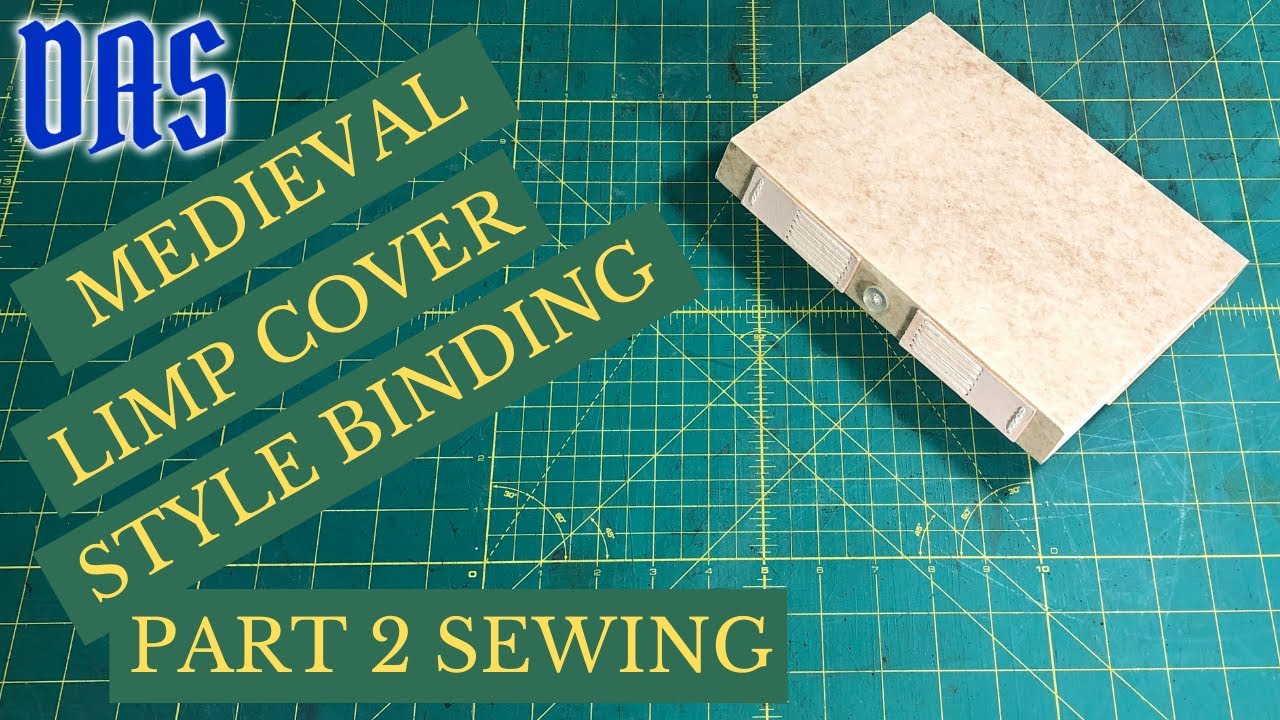The image displays a detailed cover, likely for a digital tutorial or a video. The background is primarily green, reminiscent of a quilt or material cutting mat, complete with squares, lines, angles, and various size markings in yellow. In the upper right corner, a beige, box-like rectangular object, a little darker than a manila folder, features a small pull tab. At the top left corner, bold blue letters spell out DAS, D-A-S. Along the left side, there are green strips with yellow, capitalized lettering running diagonally from the lower left to the upper right, reading "Medieval Limp Cover Style Binding." At the bottom left, another green strip simply states "Part 2 Sewing." The entire design seems to be focused on a sewing project, with elements such as a diagram or chart, emphasizing the tutorial's instructional nature.